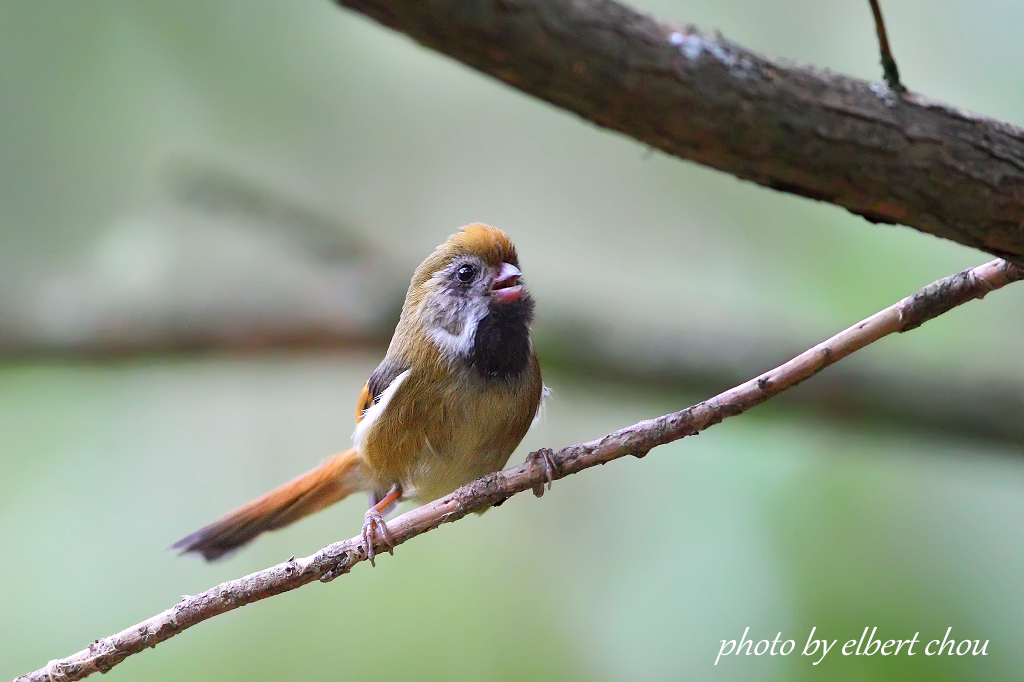This professionally shot photograph by Albert Chou features a small songbird perched prominently on a slender tree branch that extends from the bottom left to the center right of the image. The bird, centrally focused with a blurred background creating a narrow depth of field, is captured in detailed clarity. Its plumage is primarily yellow with gradients of golden tan, and it features a distinctive black spot under its neck. The bird's cheek and eyes are highlighted by a white patch, contrasting with its black eyes. It has a small, open orange beak, hinting that it might be singing or calling out. The head is orange, and its wings display a noticeable white stripe and a black spot on the shoulder. The bird’s long tail is predominantly orange, transitioning to black at the tip. There is another branch visible at the top right of the image, while the background comprises dark and light green hues, further emphasizing the bird's vibrant colors. The photograph is marked with the text "photo by Albert Chou" at the bottom right.